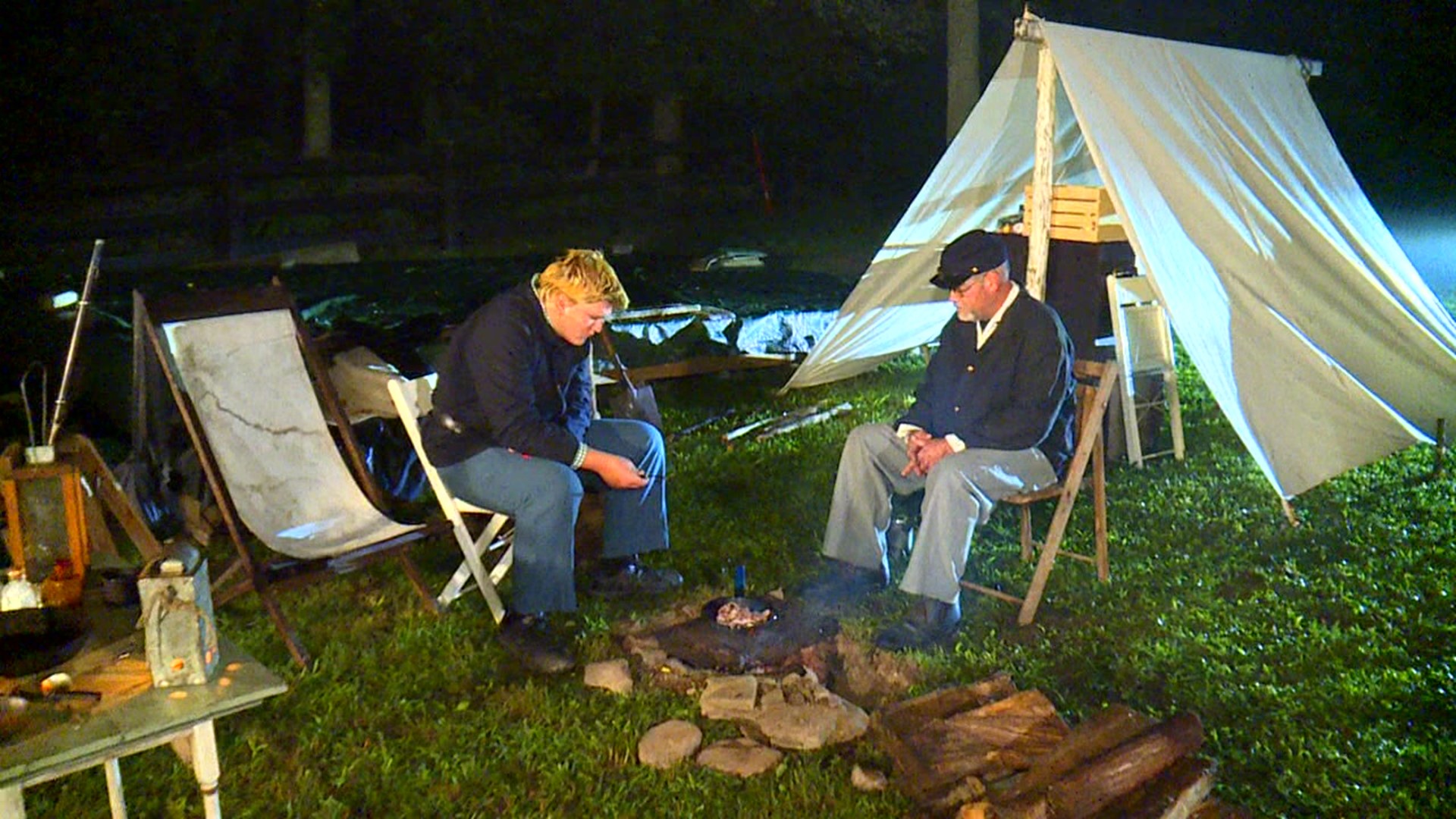This nighttime photograph captures a Civil War reenactment camp scene, featuring two men seated around a smoky campfire on a well-lit grassy area. Illuminated by nearby lights, the men are surrounded by a stack of firewood and are framed by a rustic backdrop of dark, leaf-covered trees and a dark-colored wooden fence. The individual on the left, a modern-looking man with short blonde hair, is casually dressed in blue jeans and a long-sleeve blue shirt, while seated in a chair. In contrast, the man on the right wears a Union Civil War cap, a long-sleeve blue cardigan, and gray pants, evoking a historical vibe. A rudimentary white tent, pitched with a light-colored wooden pole and appearing to store crates and other items, is positioned at the upper right of the photograph, providing additional context to the reenactment setting. The scene’s detailed ambiance offers a blend of contemporary and historical elements, brought together under the quiet, dark canopy of the night sky.